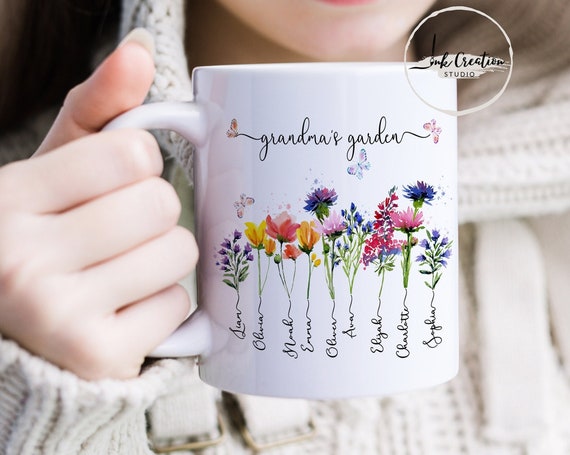This photo features a female Caucasian hand, adorned with a white wool sweater sleeve, holding a white coffee mug. The mug, from Ink Creation Studio, bears the inscription "Grandma's Garden" in elegant script. Surrounding the text are delicate paintings of various flowers, each flower sprouting from a name written in script, presumably the grandchildren's names. The names, such as Olivia and Ava, are vertically arranged, each associated with a uniquely colored bloom. The background is artfully blurred, emphasizing the detailed and personalized design of the mug. Only the woman's chin is visible, lending a warm, intimate feel to the composition.